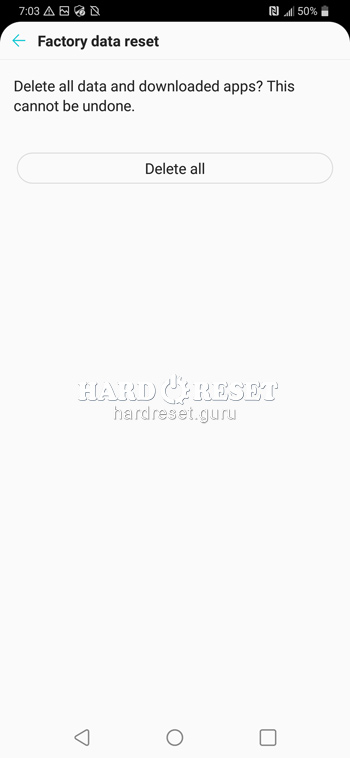The image shows a screenshot from a cell phone displaying the settings menu for a factory data reset. At the top of the screen, the status bar features a black background with white icons indicating the time is 7:03, the battery level is at 50%, and additional standard status icons are present. Below this, the background transitions to a grayish-white color. 

At the top of this section, there is a teal-colored back arrow followed by the title "Factory Data Reset" in black text. Beneath it, a warning message reads: "Delete all data and downloaded apps?" with an additional cautionary note: "This cannot be undone." Below the text, there is a prominently displayed "Delete All" button, which is long, rectangular, and has rounded edges.

In the middle of the page, there is a label in white print with a subtle border for contrast, stating "Hard Reset" with a gear icon next to it, followed by the website "hardreset.guru."

At the very bottom of the screen, the standard navigation bar features three icons: a triangle, a circle, and a square.